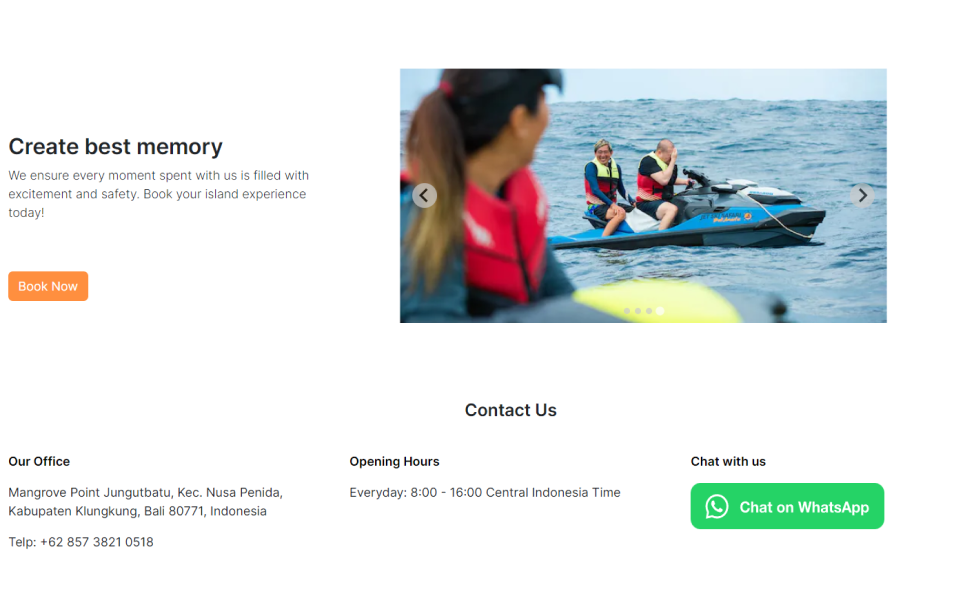The webpage features a clean design with a predominant white background and displays a small photograph in the top right corner. The heading at the top reads, "Create Best Memories," followed by a tagline that promises, "We ensure every moment spent with us is filled with excitement and safety. Book your island experience today." Below the text, there's an orange "Book Now" button inviting visitors to make a reservation.

In the top right photo, a vibrant scene unfolds with a jet ski gliding over the azure ocean. Two individuals, clad in bright yellow and red life vests, are seated on the jet ski — a man at the front and a woman at the back, both smiling and appearing to enjoy their adventure. Closer to the camera on the left side of the image, a woman with a ponytail, dressed in a red-topped life vest with a front zipper, adds a sense of engagement as she stands near the water.

Towards the bottom of the webpage, there is contact information for the office located at Mangrove Point, including the address and telephone number. Centrally placed text indicates the office's operating hours: every day from 8:00 to 16:00 Central Indonesian time. On the bottom right, there's a "Chat with Us" section, featuring a green "Chat on WhatsApp" button, providing an option for instant communication.